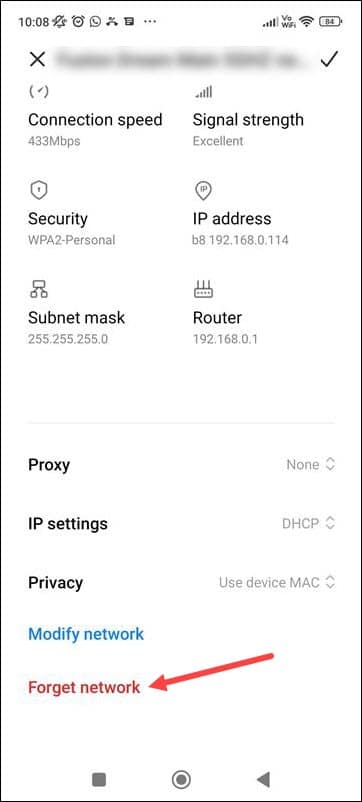This image is a detailed screenshot from a cell phone displaying various status indicators and network details. At the top-left corner, the time is shown as 10:08 AM. Adjacent to the time, there's a bell icon with a line through it, indicating that notifications are silenced. Next to the bell icon, there is a small alarm clock icon, followed by an icon depicting a phone inside a speech bubble.

On the upper-right side, the battery icon shows a charge level of 84%. To the left of the battery icon, the Wi-Fi icon is visible, indicating a connection to a wireless network, albeit with a note stating "low Wi-Fi". Additionally, the cell phone reception icon shows four out of five bars, signifying a strong signal.

Beneath these icons, there is a blurred redacted line with an 'X' icon on the left and a checkmark icon on the right. Below this line, the text "Connection Speed" is displayed with "Signal Strength" on the right. The following line reads "Security," with "IP Address" on the right. Lastly, the text "Subnet Mask" appears, with "Router" on the right-hand side.